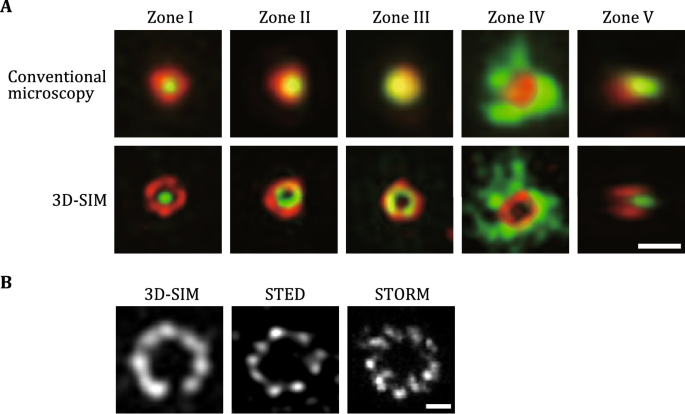The image is a detailed comparative study consisting of 13 individual square-shaped microscopic images. The top 10 images, arranged in two rows of five, are labeled "A," while the bottom 3 images form a separate section labeled "B." The top row of five images is designated "conventional microscopy," and the row immediately below it is labeled "3D-SIM," indicating a comparison between conventional microscopy and 3D structured illumination microscopy (3D-SIM).

Each set of images within the top two rows is further categorized into zones labeled 1 through 5 using Roman numerals. The images display various circular objects against a black background, featuring differences in coloration: some circles show yellow centers with red outlines, while others have red centers surrounded by green, illustrating different observation techniques.

The bottom row, labeled "B," contains three images comparing advanced microscopy techniques, specifically 3D-SIM, STED, and STORM. These images are presented in black and white, depicting white rings on a black background, which demonstrate increased resolution in microscopic imaging thanks to simulation techniques. Overall, the image showcases how different microscopic and simulation methods vary in capturing the intricate details of microscopic structures.